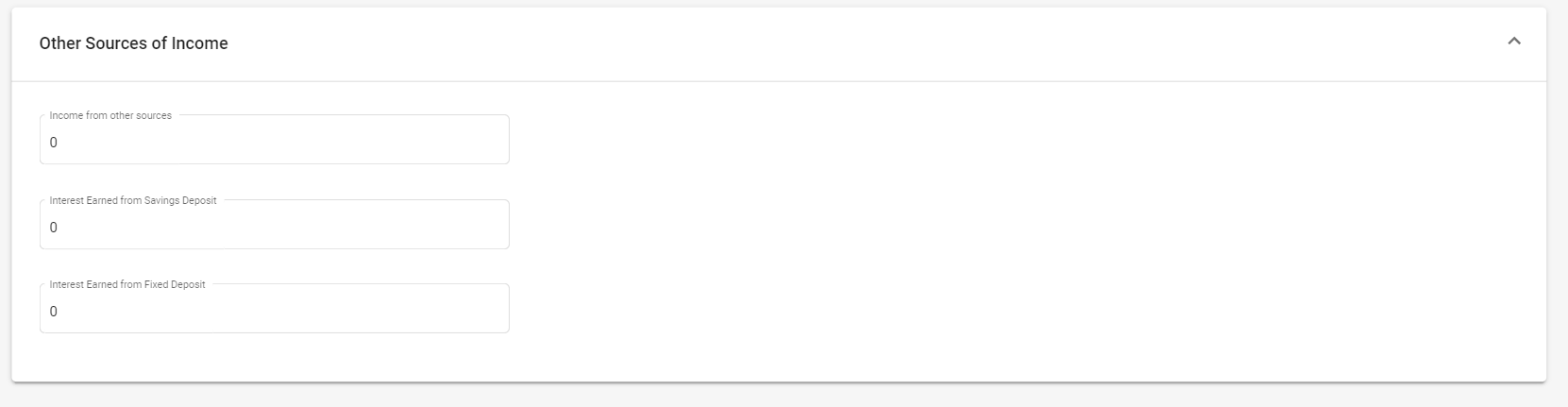The screenshot depicts a section of an unspecified website focused on financial information. The header at the top left reads "Other Sources of Income" in a dark gray font. Adjacent to this header, on the top right, is a small upward-pointing arrow icon. 

Directly beneath the header, a horizontal line spans the entire width of the screenshot, demarcating the section title from the subsequent content. Below this separator, the text "Income from Other Sources" is displayed within a light gray-bordered rectangle, showing a value of zero. 

Similarly, following this are two more entries:
1. "Interest Earned from Savings Deposit" within a gray-bordered rectangle, also showing a value of zero.
2. "Interest Earned from Fixed Deposit," again in a gray-bordered rectangle, indicating zero.

All text within these sections is in varying shades of gray, with the header “Other Sources of Income” being the darkest. The background of the screenshot is predominantly white, encased by a subtle light gray border. There is no additional text or information visible in this screenshot.